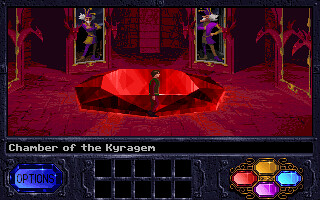In the image, there is a detailed screenshot from a video game, possibly a computer or mobile game, that depicts a medieval-themed chamber. The focal point is a man standing in the center of a room with red pyramid-like flooring and a large, radiant ruby or jewel behind him. The room is bathed in an eerie, blood-red light, giving it a mystical ambience. Various decorations adorn the chamber, including a couple of frames or tapestries featuring illustrations that resemble war art or wizards. Amidst this setting, a significant caption reads "Chamber of the Chiragim" at the bottom of the screen. Below the text, there is a blue button labeled "Options" in black lettering. Additionally, there is a row of ten square panels that might be intended to display collected items. Positioned on the far right is a set of four button-like gems in different colors arranged on a gold background, with red at 9 o'clock, gold at 12 o'clock, aqua blue at 3 o'clock, and pale purple at 6 o'clock, possibly representing a control mechanism in the game.